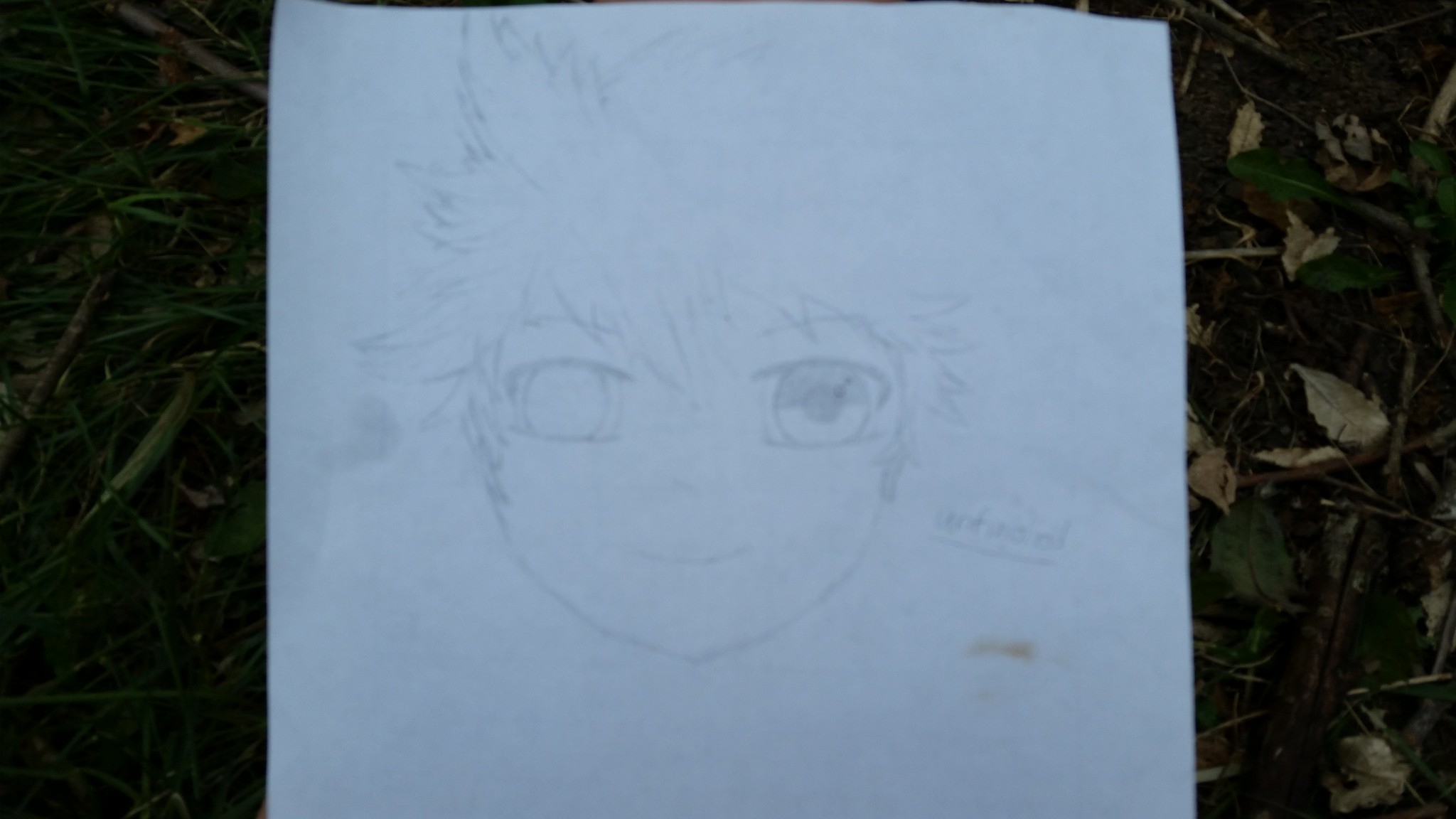This image displays a pencil drawing of an anime character on a white sheet of paper, which is lying on the ground amidst some leaves, dried grass, branches, and stems from plants, suggesting it is outdoors. The character's face is large and oval-shaped with spiky hair and jagged, uneven bangs. The eyes are exaggerated in size, characteristic of anime art: the left eye appears blank as if blind, showing only the outline of the iris, while the right eye is fully detailed with an iris and black pupil, and shaded slightly at the top. The figure's expression includes a small, curved line for a smile and a very simple, small nose made up of a couple of lines. The eyebrows are thin and black. Next to the head, there are some illegible letters and a brownish smudge at the bottom right side, along with a dark gray smudge on the center left side of the paper.